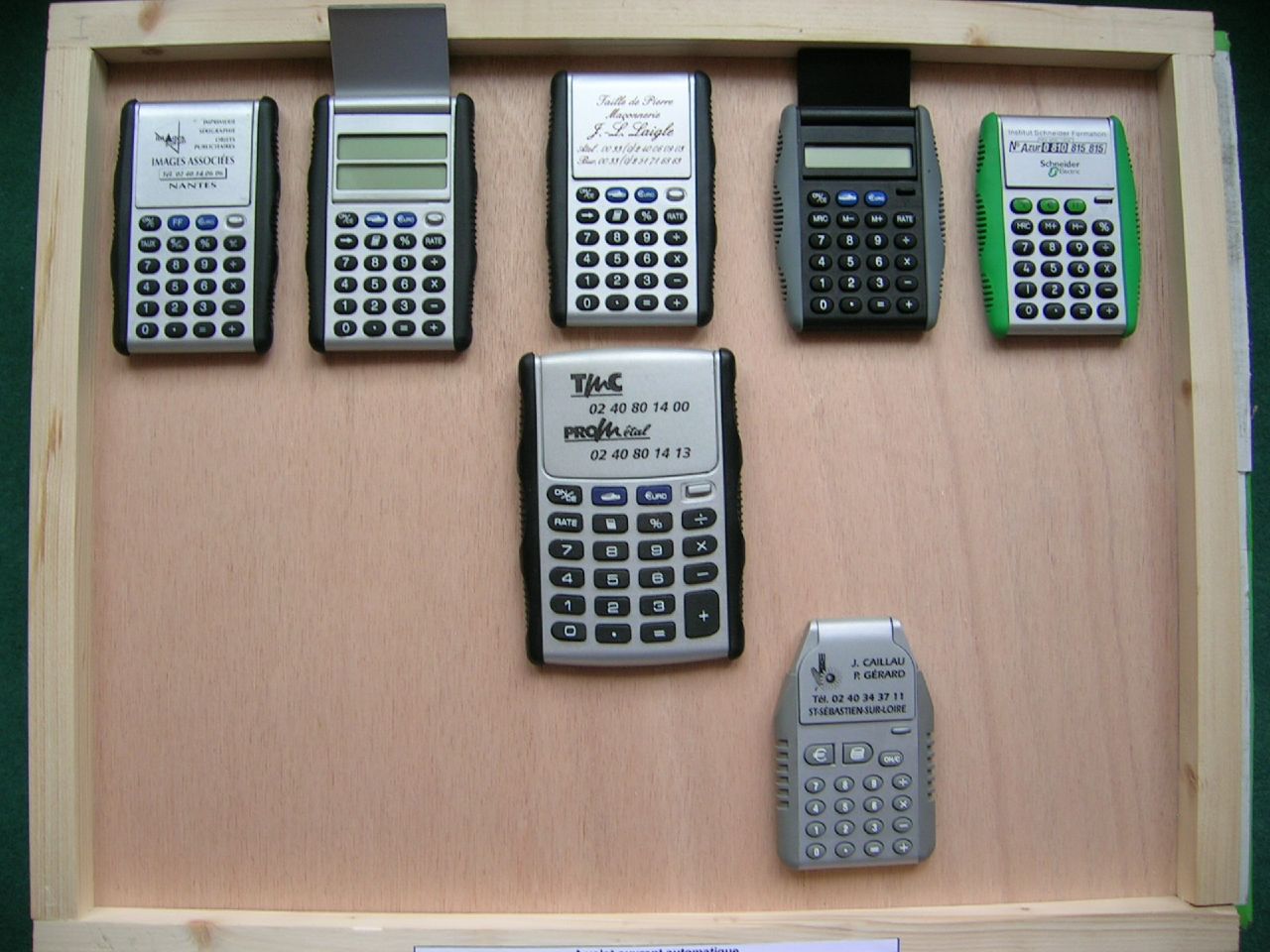This photograph features a wooden box with a light brown finish and a defined border, containing seven scientific calculators arranged in a specific layout. The calculators are largely black, gray, and silver, with some featuring additional colors and different designs. They are organized with five calculators in the top row, one in the middle, and another slightly ajar to the bottom right of the middle one. Notably, the top right calculator stands out with its bright green sides and green buttons. Brands such as TMC, Nantis, Schneider, and Images Associates are visible on some units, while others have indistinct or foreign language inscriptions. Some calculators have flaps covering the screens, with the first two identical black-and-silver models featuring ribbed sides and black buttons. The middle one of this pair has different engraving on its flap. Another notable calculator has a small upwards-turned flap revealing a blank green screen. The largest calculator, in the bottom middle, is labeled with the text "TMC-02-40-80-14-00-PRO-M-02-40-80-14-13" on its flap. These details collectively highlight the variety and uniqueness of the calculators within the wooden container.